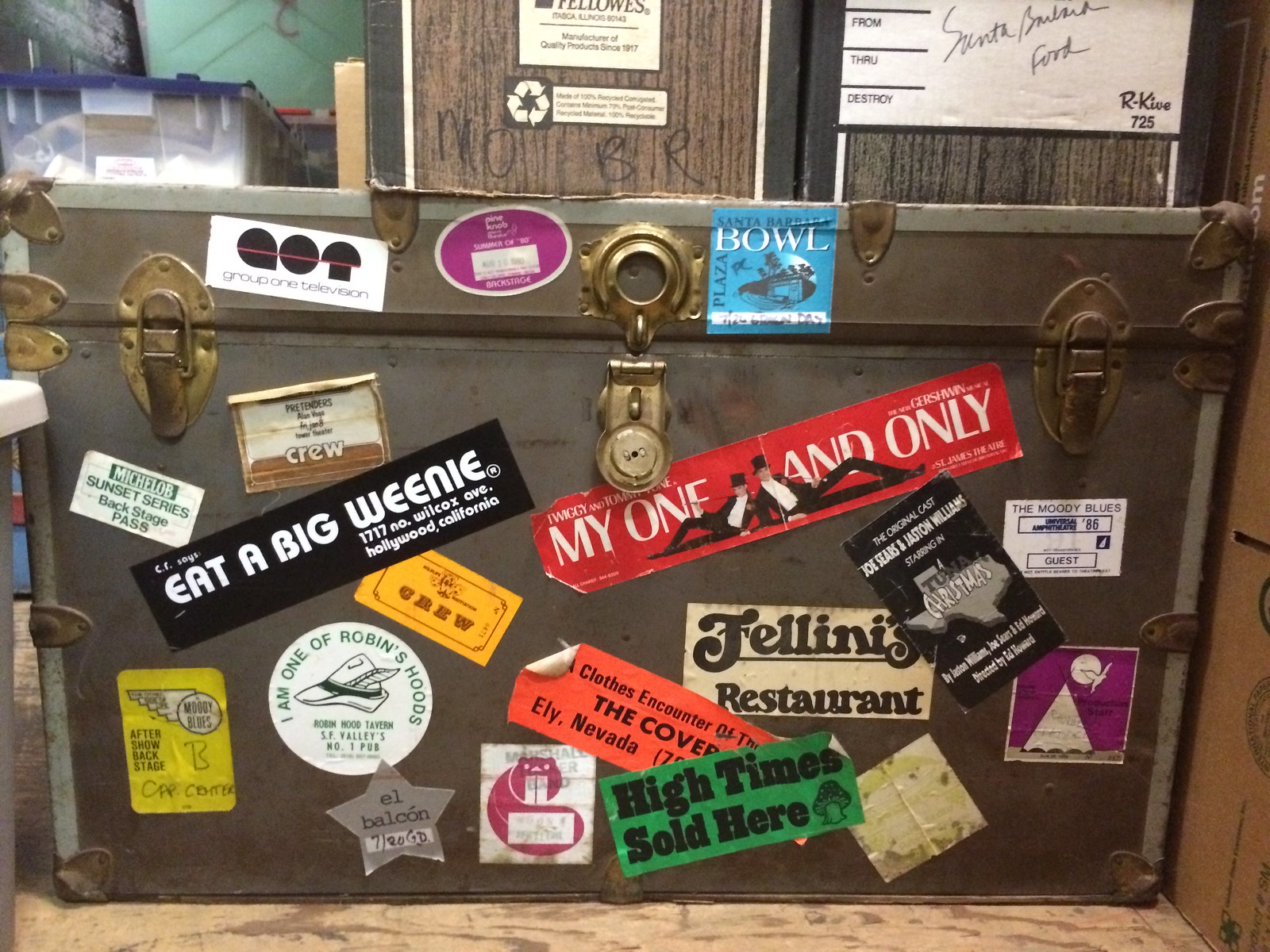The photograph captures an old-fashioned steamer trunk, prominently positioned on a wooden floor. The trunk appears silver-gray with a slightly rusted, worn look and features gold locks and clasps, although the middle latch hangs loose. It is adorned with a variety of colorful and worn stickers, some with curled edges from age and wear. Notable stickers include a large, red one reading "My One and Only" with the image of two men in tuxedos and top hats; a green sticker with black text and a mushroom that says "High Time Sold Here"; and a black sticker with white writing that reads "Eat a Big Weenie, 1717 Wilco Ave, Hollywood, California." There’s also a noticeable white sticker with a pink silhouette of a cat and a silver star-shaped one that says "El Balcón." Additional stickers in various shapes and colors—yellow, blue, purple, and more—add to the trunk's eclectic appearance. In the background, there are old-looking filing boxes stacked and a Tupperware type plastic storage container with a blue lid to the left.